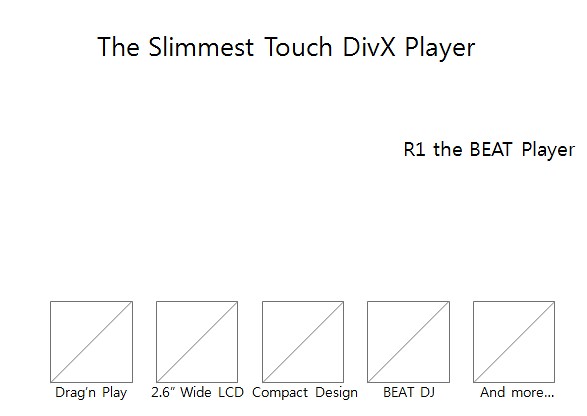The image appears to be either an advertisement or setup screen for a DivX-type DVD player. The design is minimalist, with black text on a white background. At the top, the text reads "The Slimmest Touch DivX Player." Below and slightly to the right, it states "R1, The BEAT Player," with "BEAT" in capitals. Under this header, there are five identical squares, each containing a diagonal line from the bottom left to the top right corner, resembling two triangles stacked together to form a square. These squares serve as icons with accompanying text descriptions: "Drag 'n Play" under the first, "2.6 inch wide LCD" under the second, "Compact Design" under the center square, "BEAT DJ" in all capitals under the fourth, and "and more..." under the final square. The entire presentation is black and white, with the icons and text arranged in a straightforward, easy-to-read format.